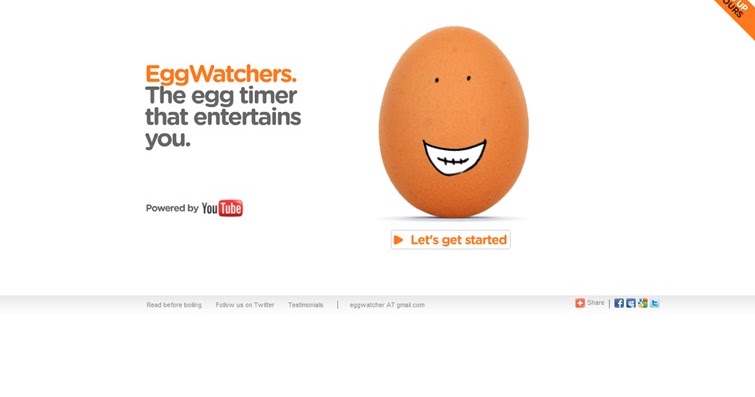This is a still image that likely serves as the introduction to a YouTube video. At the center of the image is a drawing of a brown egg, adorned with two small black dots for eyes and a white, black-outlined mouth giving it a whimsical face. To the left of the egg, the text "Egg Watchers" is prominently displayed in orange, followed by the tagline "The egg timer that entertains you" written in dark blue. Beneath this, in blue text, the phrase "Powered by" is followed by the YouTube logo, where "You" is in blue and "Tube" is encased in a red rectangle.

Just below the egg, there is a call-to-action statement in blue text: "Let’s get started," accompanied by an orange arrow suggesting where to click to commence the video. Further down, additional instructional and contact information is provided: "Read before boiling," "Follow us on Twitter," "Testimonials," and an email contact "eggwatcher@gmail.com." There is also a "Share" button with a plus icon, alongside social media icons for Facebook and Twitter.

Altogether, this image sets the stage for an engaging YouTube video, capturing attention with its playful design and clear instructions.